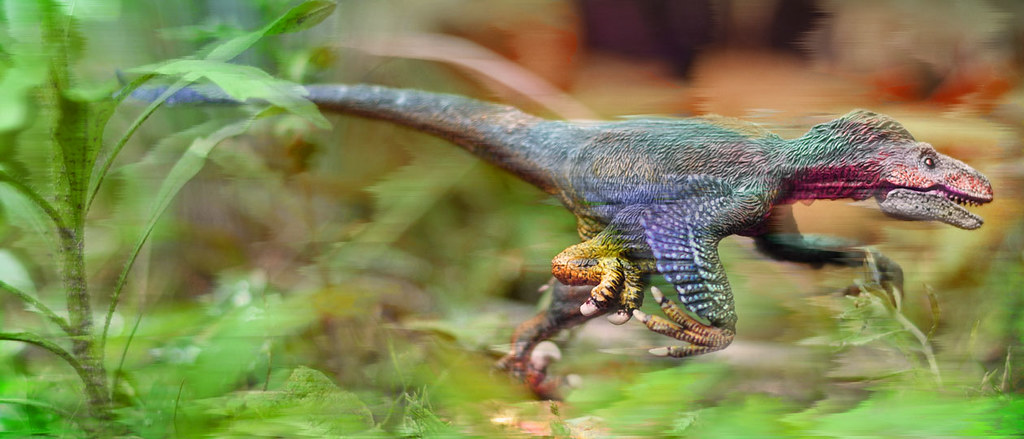The image depicts a dynamic side profile of a dinosaur, resembling a velociraptor, running to the right with a blurred backdrop suggesting high-speed motion. The dinosaur combines lizard-like and bird-like features; it has gray scaly skin with notable red markings around its mouth and neck, and feathers on its forelimbs and back. The creature's mouth is open, showcasing tiny teeth, and its dark eyes are focused forward. Its back right leg displays some yellow scales, and the right front leg is in mid-air, emphasizing the rapid movement. The leg extends with long claws, each tipped with sharp nails. The background transitions from tall green weeds on the left to flat green grass, with the majority of the image being an out-of-focus blend of green hues, heightening the sense of motion. A tall leaf stalk curves outward on the left side, contrasting with the blur that defines the scenery, making the dinosaur the primary focus of the composition.